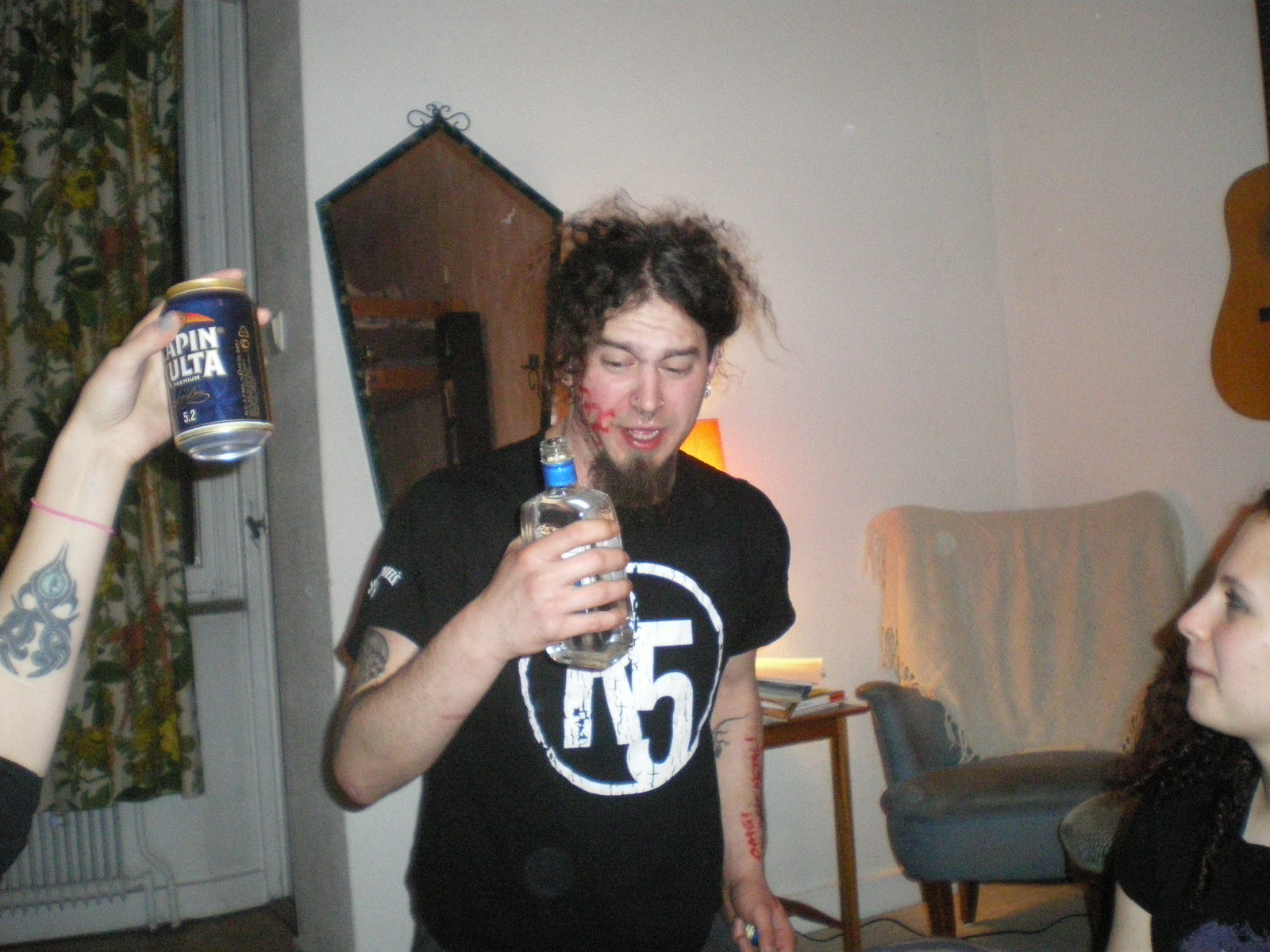This photograph captures an energetic, fun-filled house party attended by young adults. In the center of the scene, a bearded male wearing a black t-shirt emblazoned with a logo resembling "R5" smiles with his mouth open, eyes partially shut, holding a clear bottle of alcohol, likely vodka. His curly hair is partially tied back, and he has red markers or tattoos on his face and arm, possibly indicating party shenanigans like being graffitied while drunk.

To the left, a woman dressed in a black sweater with sleeves pushed past the elbows extends her arm, showcasing a tribal or mask tattoo on her forearm. She holds a beer can that reads "Apenolta," and wears a thin white or red bracelet on her pale skin. Her face isn't fully visible in the photograph. 

In the lower right corner, a woman with long brown hair partially obscures her face as she looks towards the man in the center. She too is dressed in a black t-shirt.

The background details a cozy living room setting with various elements: a guitar mounted high on the wall, a mirror, a doorway leading to another room, a window with a curtain, an easy chair draped with a blanket, and a table cluttered with books, magazines, and a lamp. This scene encapsulates the lively, youthful atmosphere of a typical party among twenty-somethings.